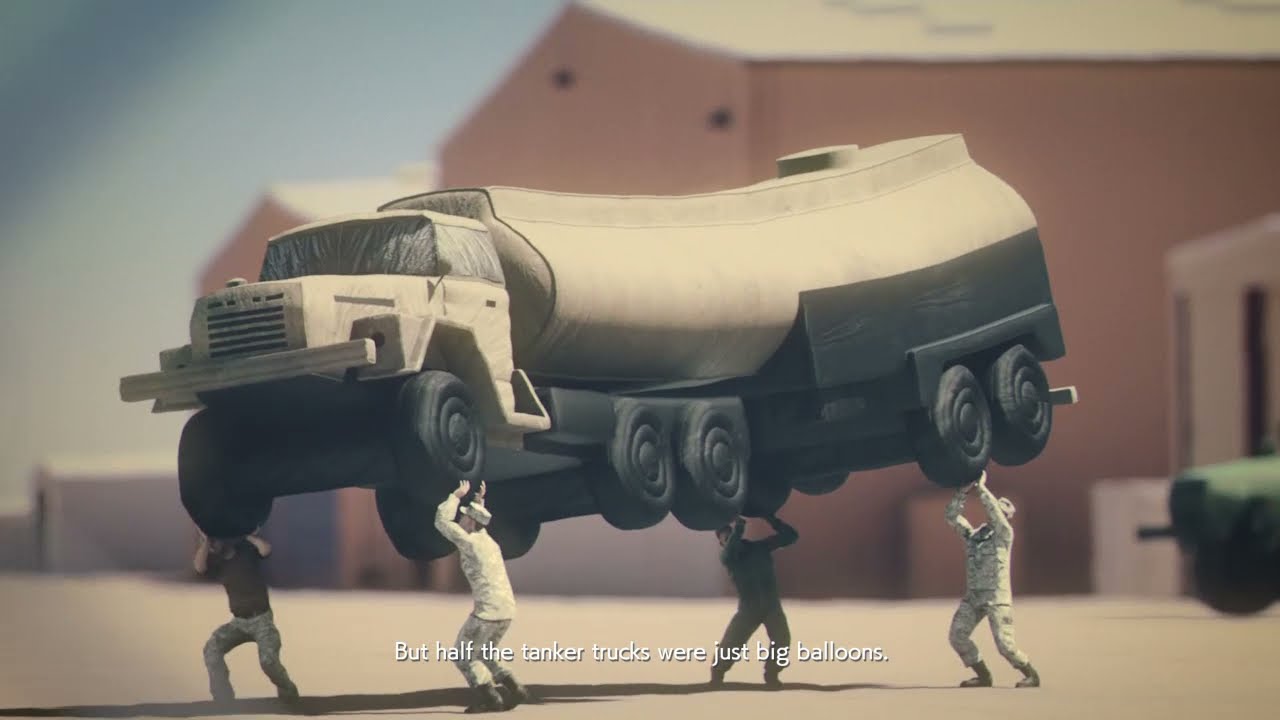In this highly detailed digital artwork, a wide rectangular image captures an intricate scene that blends elements of realism and artistic stylization. Central to the composition are four men, each stationed at a corner, seemingly lifting a tanker truck with black wheels and a tan-colored, curved body. The truck appears to sag in the middle, giving the impression that it is made of a soft material, perhaps a balloon, as suggested by the text at the bottom that reads, "but half the tanker trucks were just big balloons." The men are dressed in various outfits, including camouflage and long sleeves, with one sporting green pants and a blue shirt, while another at the front, on the passenger side, wears a brown shirt. 

In the background, a towering, reddish-brown building with a light yellow triangular roof dominates the right and middle sections of the image. Behind it to the left, a smaller but similarly styled structure peeks out. A blurry gray wall also appears in the distant background. The left side of the image reveals a sky gradient, light blue transitioning to darker hues toward the corner. The ground in the foreground is light yellow, presumably a parking lot, setting the stage for this dynamic and vividly detailed scene.